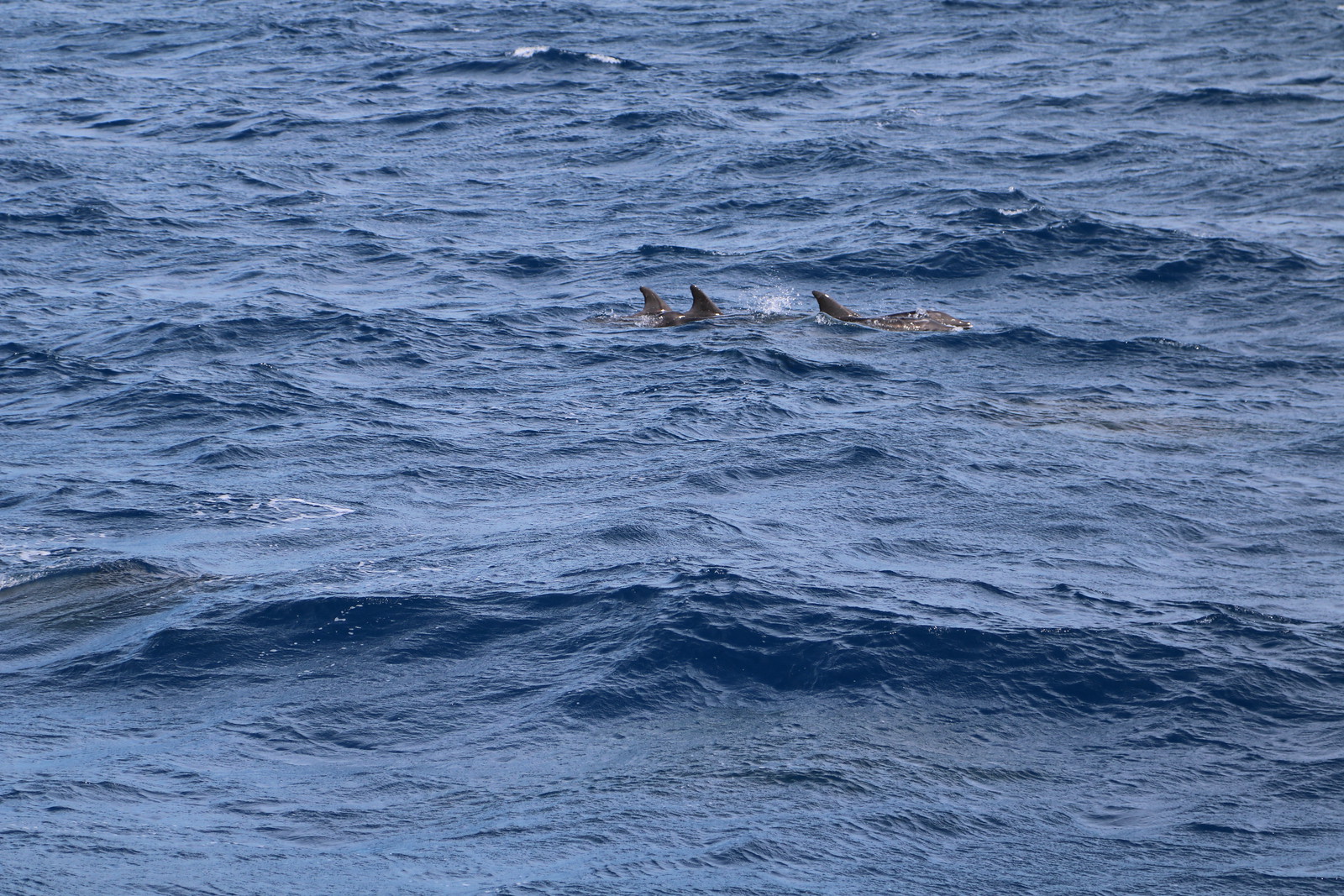The photograph captures a mesmerizing daytime ocean scene with deep, navy blue water marked by gentle ripples and occasional small white caps, indicating a slightly choppy day. Centrally located in the frame are the distinctive dorsal fins of three marine animals—likely dolphins or sharks—appearing in a staggered line as they swim towards the right. The leading fin reveals a glimpse of a dark gray or black body just beneath the surface, while the other two fins are primarily exposed above the water. The sunlight illuminates the entire scene evenly, ensuring the image is well-focused and brilliantly lit without noticeable shadows. The water’s serene, undisturbed stretches contrast with the lively appearance of the fins, creating a dynamic and engaging snapshot of oceanic life.